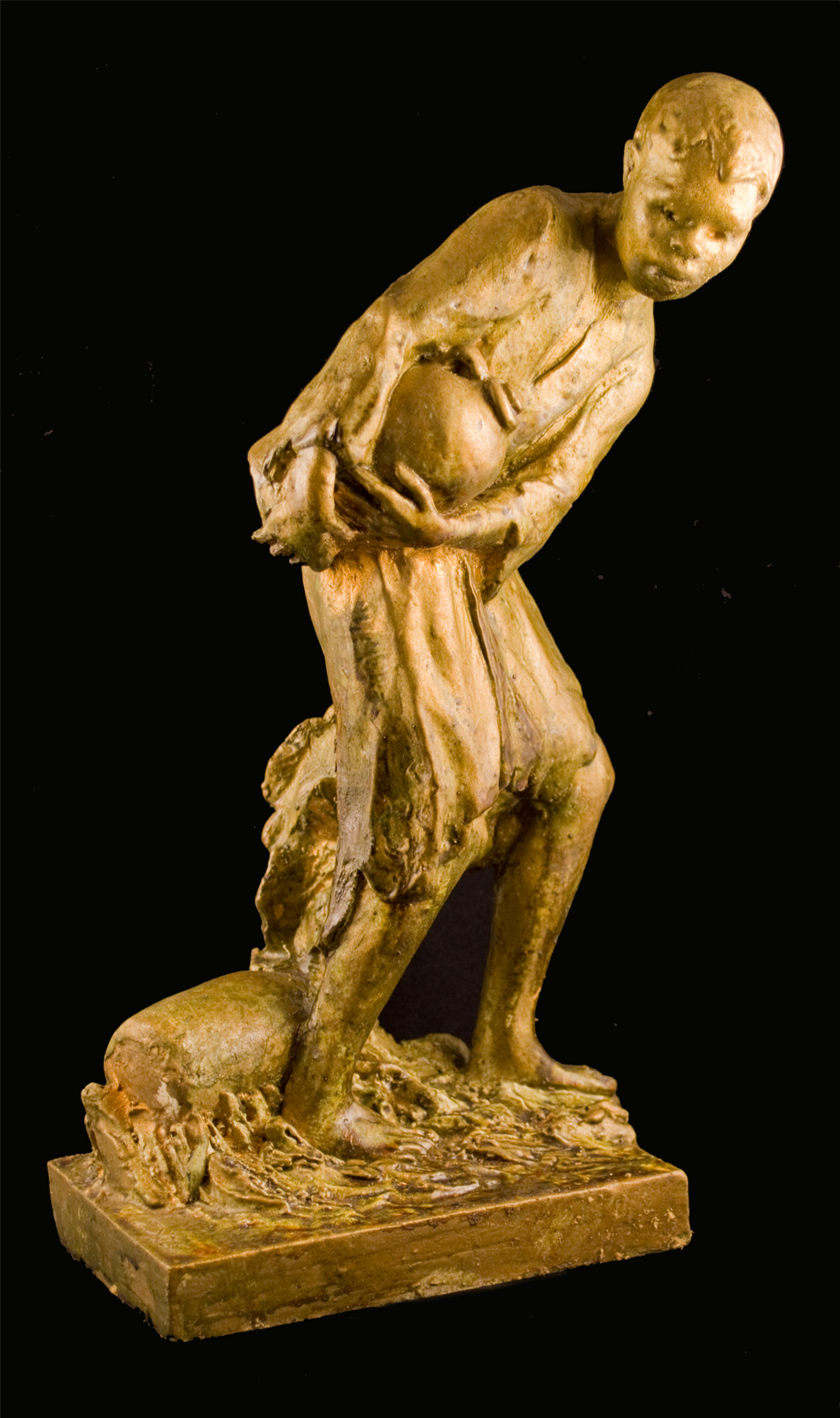This image showcases a detailed sculpture of a young African American boy, approximately 9 or 10 years old, standing prominently in the center against a stark black background. The sculpture, rendered in hues of gold, bronze, light brown, yellow, and orange, depicts the boy slightly bent forward with knees slightly flexed, his gaze directed downward towards his right foot. He is barefoot and stands on a rectangular platform that combines both golden and wooden tones. The boy appears to be holding a spherical object—perhaps a ball, vase, or pot—with both hands. His attire is tattered, adding a sense of realism and depth to the sculpture. Additionally, there is a cylindrical object behind one of his legs, and various indistinct items scattered on the ground around him. This evocative piece, reminiscent of an artist's creation suited for a museum display, captures a poignant moment with meticulous detail.